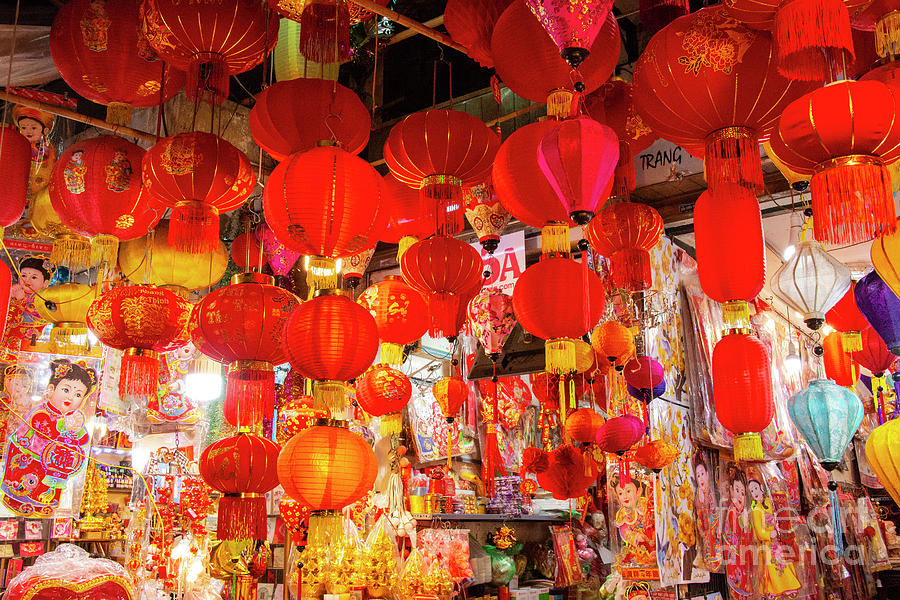This captivating image showcases a bustling shop filled with vibrant decorations, creating a festive atmosphere reminiscent of the night markets in Hanoi or a lively street in Chinatown, possibly in China, Thailand, or Vietnam. Dominated by the color red, the scene is adorned with an impressive array of over 50 red silk lanterns of various sizes, some hanging higher than others, interspersed with lanterns in white, blue, yellow, and purple hues. These lanterns come in different shapes, including oval and cylindrical. The shop is likely preparing for a celebration, possibly Chinese New Year, given the abundance of red, a color symbolizing good luck. To the left, there are numerous gold ornamentations and decorations for sale. At the bottom, baskets filled with candies or confections add to the festive spirit. A small watermark in the bottom right corner reads "Fine Art America," subtly blending into the vibrant scene.